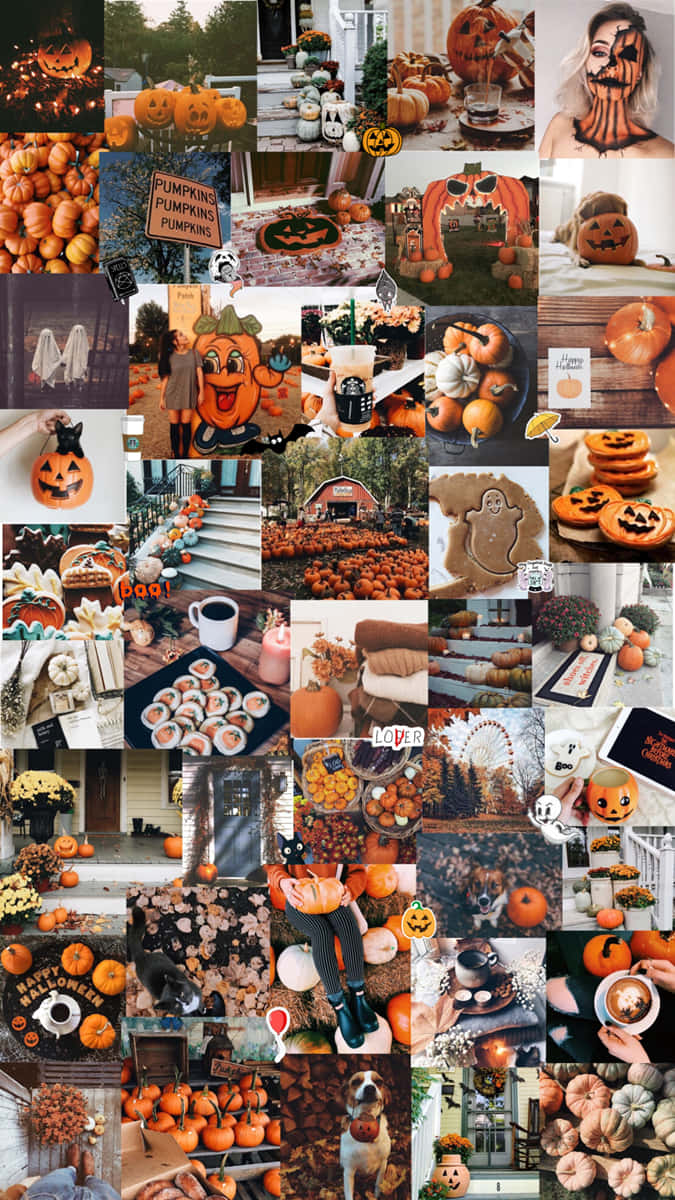This collage consists of 45 distinct images, each dedicated to a Halloween theme. The images vary, some depicting people while others showcase pets, all embodying the essence of Halloween. The scenes are a mix of indoor and outdoor settings, with the outdoor shots capturing the vivid colors of fall. Nearly every image includes pumpkins in some form—whether it's pumpkin cookies, a pumpkin sign, a pumpkin-themed doormat, or even an elaborate pumpkin arch at a Halloween festival. Among the photos, you'll find an array of Halloween elements, from intricately carved jack-o'-lanterns and spooky ghost decorations to festive Halloween masks, makeup, and themed food items. The collection offers a comprehensive visual celebration of Halloween traditions and festivities.